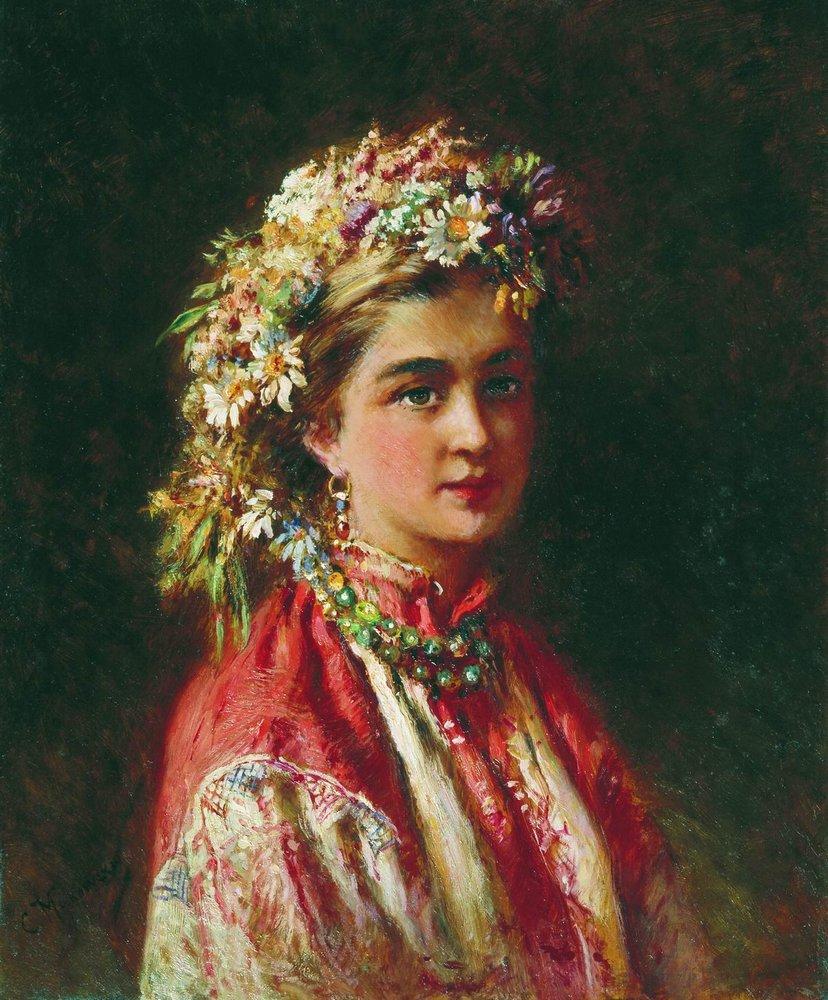This image features a detailed painting of a young woman, positioned centrally, almost directly facing the camera. The background is predominantly dark, with hints of multicolored hues that provide a subtle yet rich contrast to the subject. The woman, seated and seen from about the waist or chest up, is depicted wearing a richly elaborate red dress or jacket with lighter colored sleeves and intricate ornamentation in blue and cream around the shoulders. Her blonde hair is adorned with an array of flowers including white daisies, purple, pink, and field flowers, forming a crown of sorts. Large, dark eyebrows accentuate her expressive face, along with her red lips and noticeable dangled earrings featuring a gold structure and red beads. Around her neck, she wears a colorful bead necklace, primarily green, with additional red and yellow beads. The painting's style and detailed composition suggest it could be seen hanging in a gallery or a museum, reflecting a sophisticated piece of portraiture art.